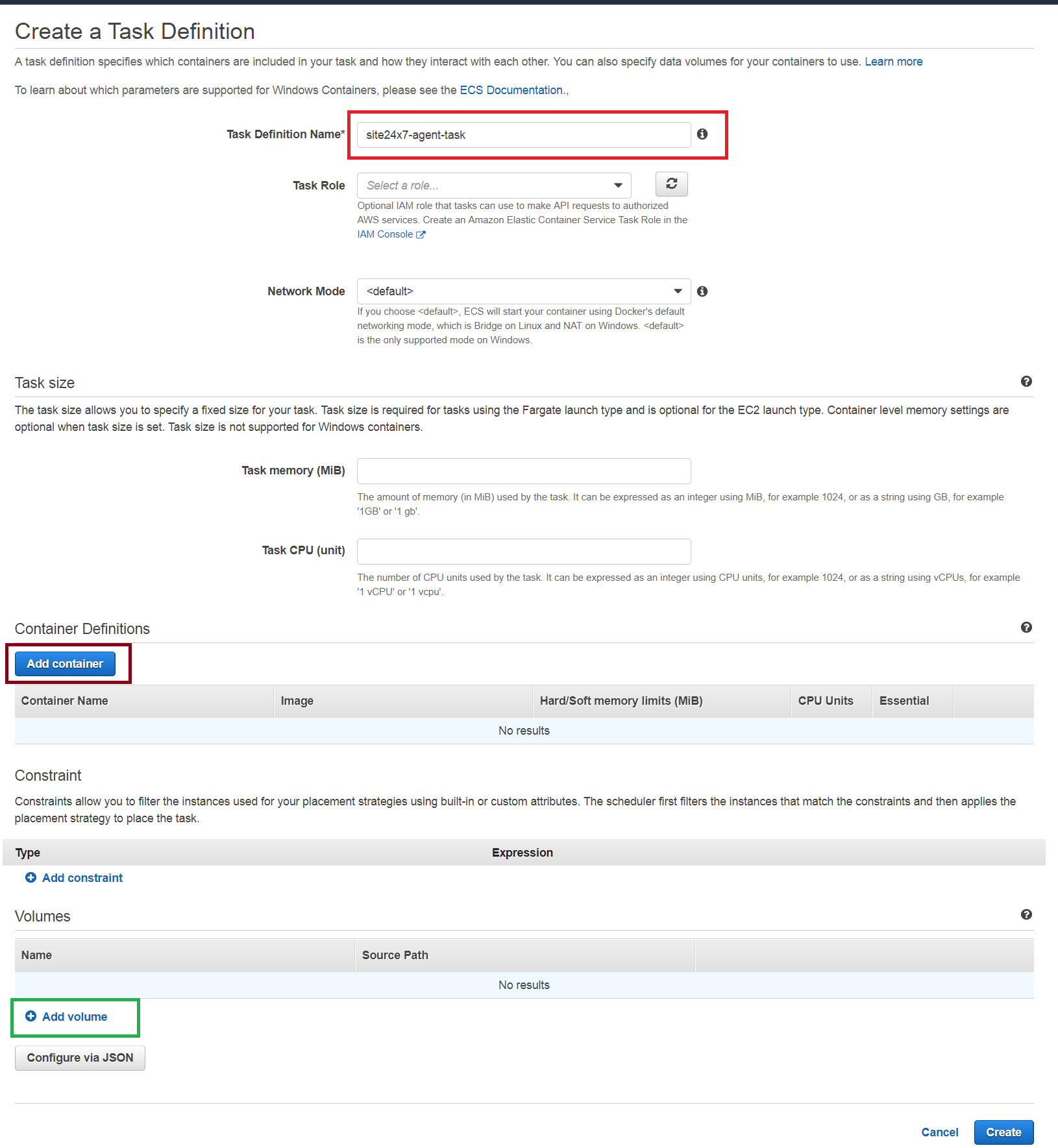**Detailed Caption:**

In the user interface of a web application for creating a task definition, the top section features a slim black bar. Below this bar, the header "Create a Task Definition" is prominently displayed. The subsequent section reads: "A task definition specifies which containers are included in your task and how they interact with each other. You can also specify data volumes for your containers to use." A blue hyperlink labeled "Learn More" follows this description.

Further down, a prompt in blue text advises users: "To learn about which parameters are supported for Windows containers, please see the ECS Documentation," with "ECS Documentation" also acting as a clickable link.

The next section is organized into various input fields and settings for the task definition, beginning with a red-circled input box for the "Task Definition Name." Under this, the "Task Role" field appears, accompanied by some semi-visible instructions. The "Network Mode" setting follows, presented alongside an explanatory note.

To the left, a gray bar titled "Task Size" introduces input fields for task configuration, including "Task Memory (MB)" and "Task CPU," each with additional information beneath.

Another categorically structured section appears next, labeled "Container Definitions," introduced by a gray bar. This section includes a prominent blue "Add Container" button, highlighted with a red circle. Detailed input fields within it allow users to define various parameters like "Container Name," "Image," "Memory Limits" (hard and soft), "CPU Units," and whether the container is essential or not. Below, a blue "No Results" message indicates the current lack of entries.

The "Constraints" section follows, partitioned by another gray bar, with sections for "Type" and "Expressions," as well as an "Add Constraints" button in blue.

Finally, the "Volumes" section is introduced by a gray bar, with headers "Name" on the left and "Source Path" towards the center. A light blue bar signals "No Results," and to the left, a green-circled "Add Volume" button awaits user interaction. A small button marked "Configure via JSON" sits above the final gray bar at the bottom of the page.

Concluding the interface, on the left of the bottom gray bar, are "Cancel" and "Create" buttons for finalizing or discarding the task definition.